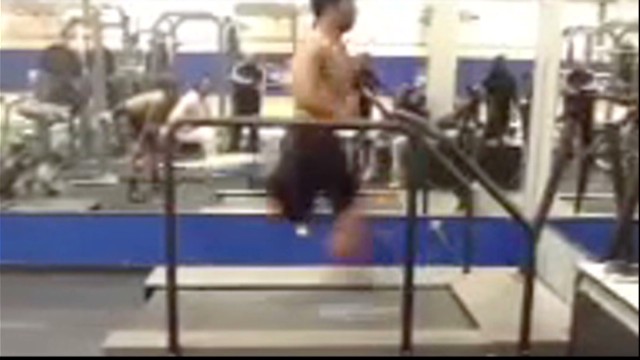The image depicts a very blurry scene inside a gym, with the central focus being a shirtless gentleman who appears to be running on a treadmill at high speed. His legs are so blurred, they almost seem to vanish, giving the illusion that he is floating in mid-air. Surrounding him are various gym machines and equipment, with the ground possibly being either hard or padded, although it's difficult to discern due to the poor image quality. In the background, a mirror reflects the interior of the gym, showing about three or four other men who are either working out or standing near weight equipment, all similarly blurred. The colors in the image include shades of white, black, gray, silver, blue, yellow, brown, and tan. Despite the blurriness, the central figure is positioned almost exactly in the center of the frame, within what seems to be an indoor gym setting, presumably taken in the middle of the day.